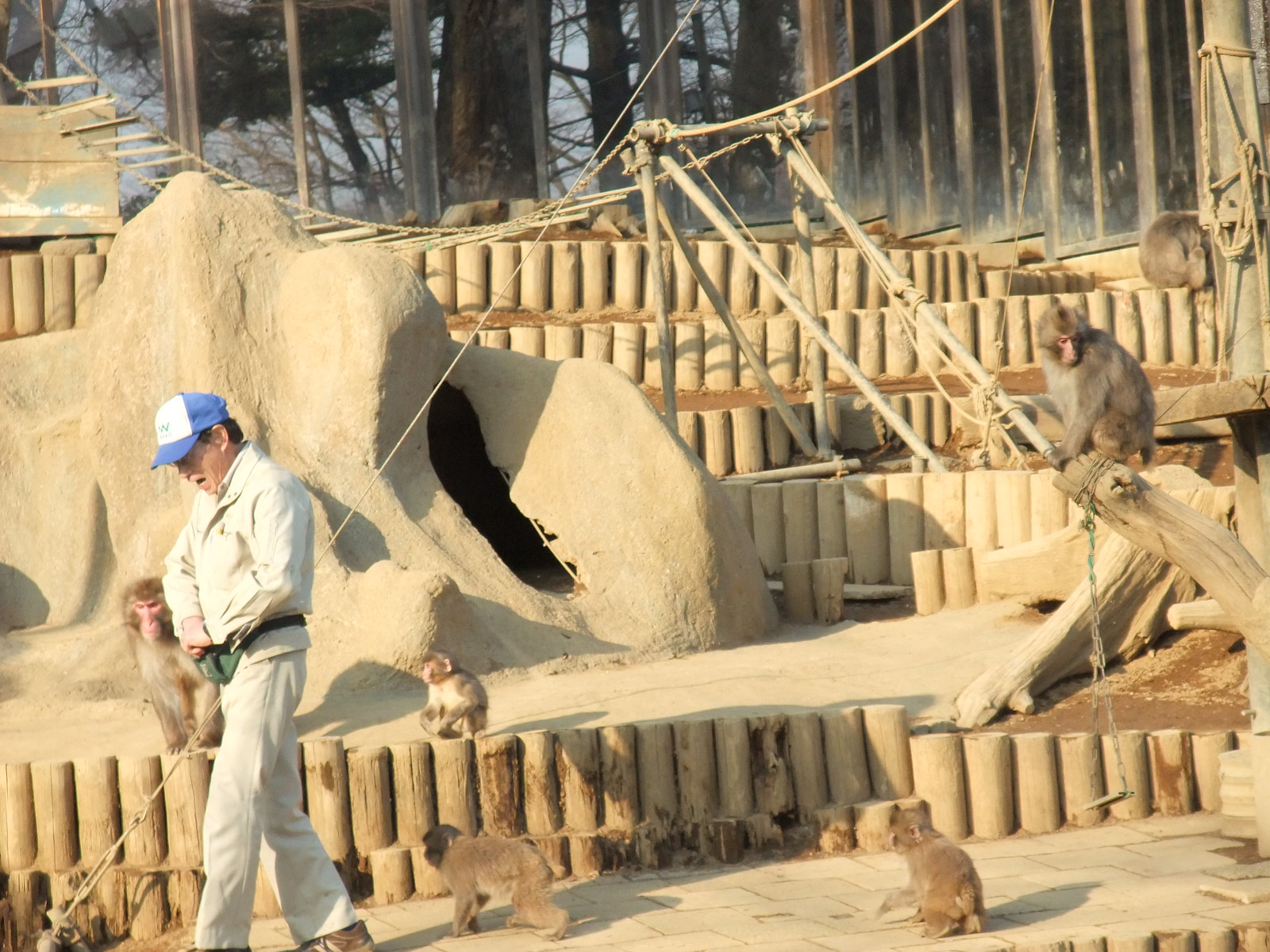In this detailed and immersive zoo scene, a man dressed in a khaki uniform, consisting of a beige button-down shirt, beige pants, and brown shoes, is prominently featured walking in a monkey enclosure. He is also wearing a blue and white baseball cap and has a green fanny pack from which he appears to be retrieving something, mouth slightly open as if speaking. Surrounding him are at least six monkeys of varying sizes, exhibiting a light grayish-brown coloration. The backdrop of this enclosure includes an assortment of tiered structures, wooden stumps arranged in rows, bamboo log fences, and various concrete surfaces. In the center, a prominent beige sandstone rock formation with a cave-like recess is visible, suggesting a resting spot for the animals. The setting exudes a naturalistic feel with dark tree trunks and branches scattered throughout and some trees at the perimeter. High above, a rope ladder with wooden steps and other playful perches are suspended, integrating with the habitat designed for the monkeys. One of the monkeys is perched on a branch in the upper right-hand corner, while others are either sitting on logs, ledges, or walking around the enclosure.